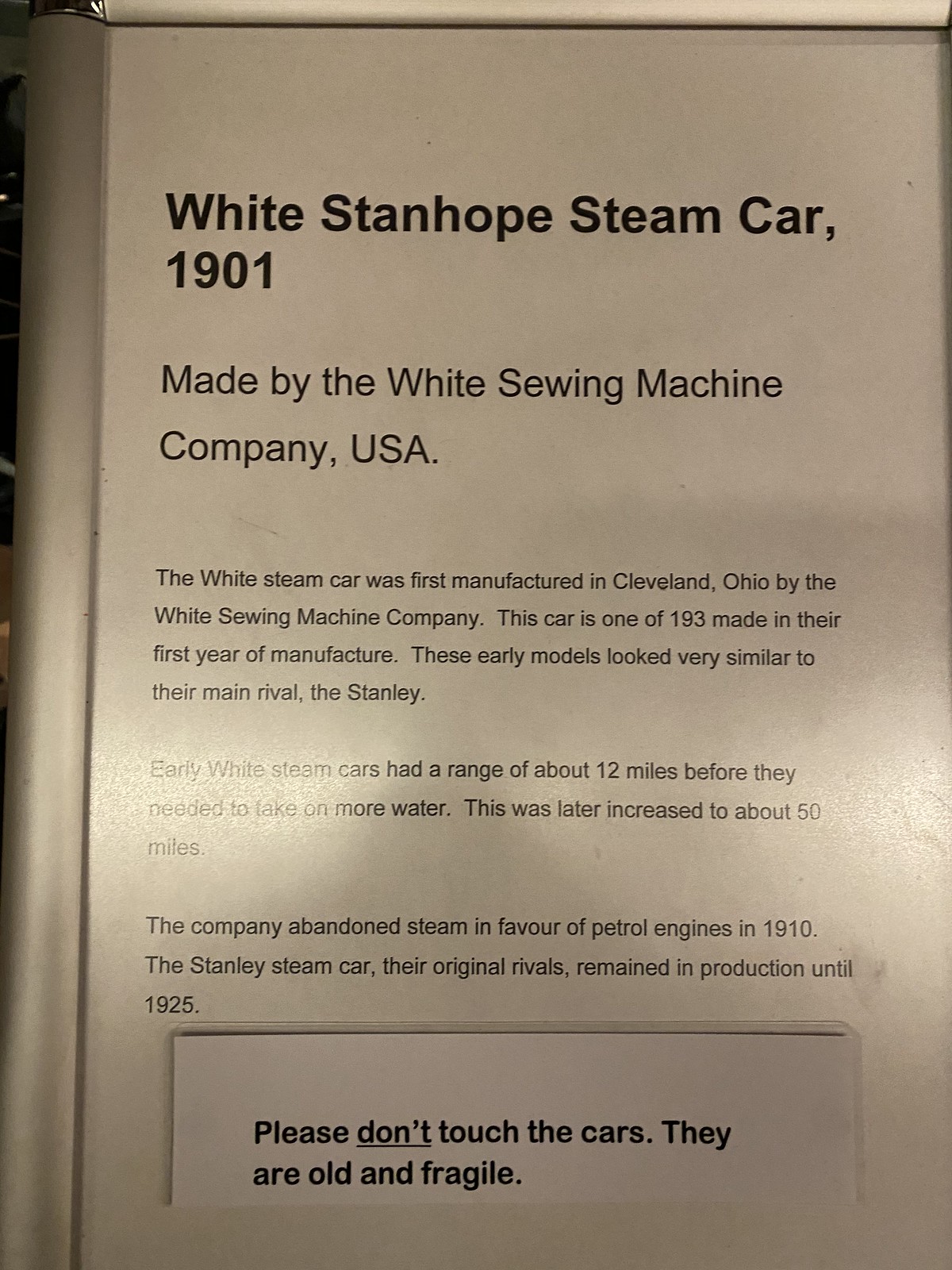This is a detailed display placard from a museum exhibit about the White Stanhope Steam Car from 1901, created by the White Sewing Machine Company, USA. The background is white with black text, suggesting it might be laminated or behind glass due to a white glare in the middle third. The placard is framed with a metal side. The topmost, bold text reads "White Stanhope Steam Car, 1901," followed by medium-sized text, "Made by the White Sewing Machine Company, USA." Below this, a detailed description spans several paragraphs:

"The White Steam Car was first manufactured in Cleveland, Ohio by the White Sewing Machine Company. This car is one of 193 made in their first year of manufacture. These early models looked very similar to their main rival, the Stanley. Early White Steam Cars had a range of about 12 miles before needing more water, later increased to about 50 miles. In 1910, the company abandoned steam engines in favor of petrol engines. The Stanley Steam Car, their rival, remained in production until 1925."

At the bottom of the placard, a printed notice says, "Please don't touch the cars. They are old and fragile."